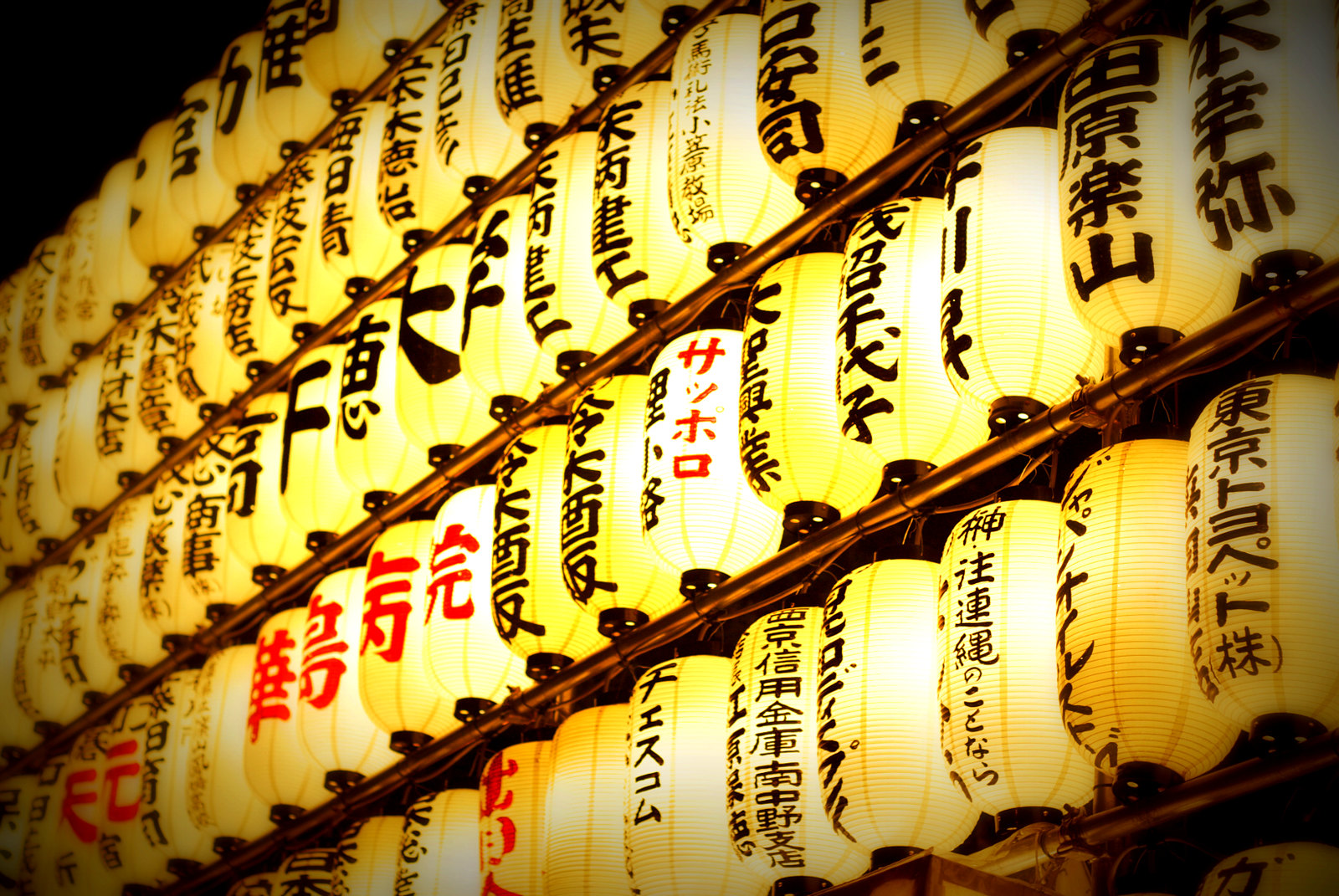The photo showcases a close-up view of a striking display of Japanese lanterns arranged in five neat rows. Each lantern radiates a warm, yellow glow from its internal light source, highlighting its translucent paper or fabric surface. The lanterns, uniformly about 12 inches tall and 6 inches in diameter, hang from an unseen structure, possibly metal bars, and are supported by shelves or wooden framework. The characters on the lanterns vary, with most featuring bold black lettering and a few adorned with red symbols. Some lanterns display a single Japanese character, while others have multiple vertically aligned symbols. The uppermost row predominantly features stark black lettering. The photograph, taken at an angle, emphasizes the organized pattern and the vibrant, illuminated atmosphere, creating a captivating visual of traditional Japanese lantern artistry.